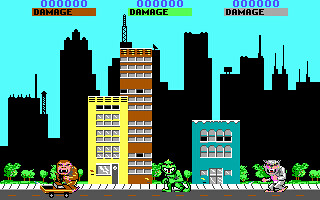This is a detailed caption of a small video game screenshot. 

The image captures a vibrant urban scene dominated by three distinct buildings. To the center-left, there is a rectangular yellow building with four levels. Each level features three glass panes, and there is a small gray door at the base. Directly beside it stands a tall rectangular brown building consisting of twelve levels, each level adorned with four horizontally-aligned windows. Towards the right, a smaller blue building with three levels can be seen, featuring two levels of four windows each, all adjacent to a sidewalk.

In the foreground, three anthropomorphic characters are displayed, each representing different animals. On the left, a monkey is riding a skateboard. In the center stands a green monster. On the right, there is a whitish monster. All three characters seem to be ready for action.

The background reveals a cityscape silhouette with various skyscrapers, etched in black against a light blue sky. At the top of the screen, health or damage meters are visible: a brown meter for the monkey on the left, a green meter for the green monster in the center, and a purple meter for the whitish monster on the right.